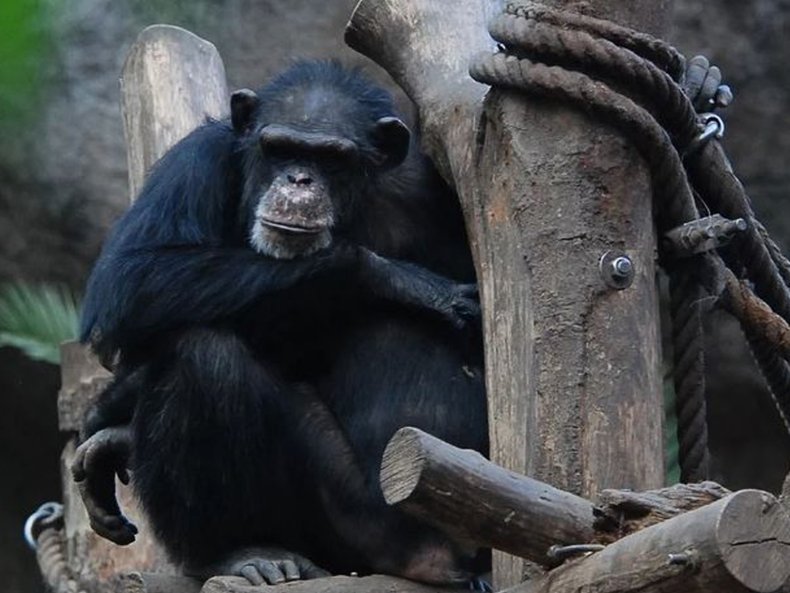The image features a fully-grown chimpanzee seated on a man-made wooden structure, likely within a zoo enclosure. The structure consists of several sawed-off logs fastened together with bolts and washers, and features heavy-duty ropes attached with metal brackets. The chimpanzee, covered in black fur with a slightly gray face, is positioned between two prominent logs. It has its knees up and arms folded, with its right arm leaning on its knee and its left arm wrapped around a log while touching one of the ropes. The background shows blurred green foliage, including an identifiable fern to the left of the chimpanzee. The scene appears to be captured in daylight, highlighting the relaxed posture of the chimpanzee, which gazes slightly to the left of the camera.